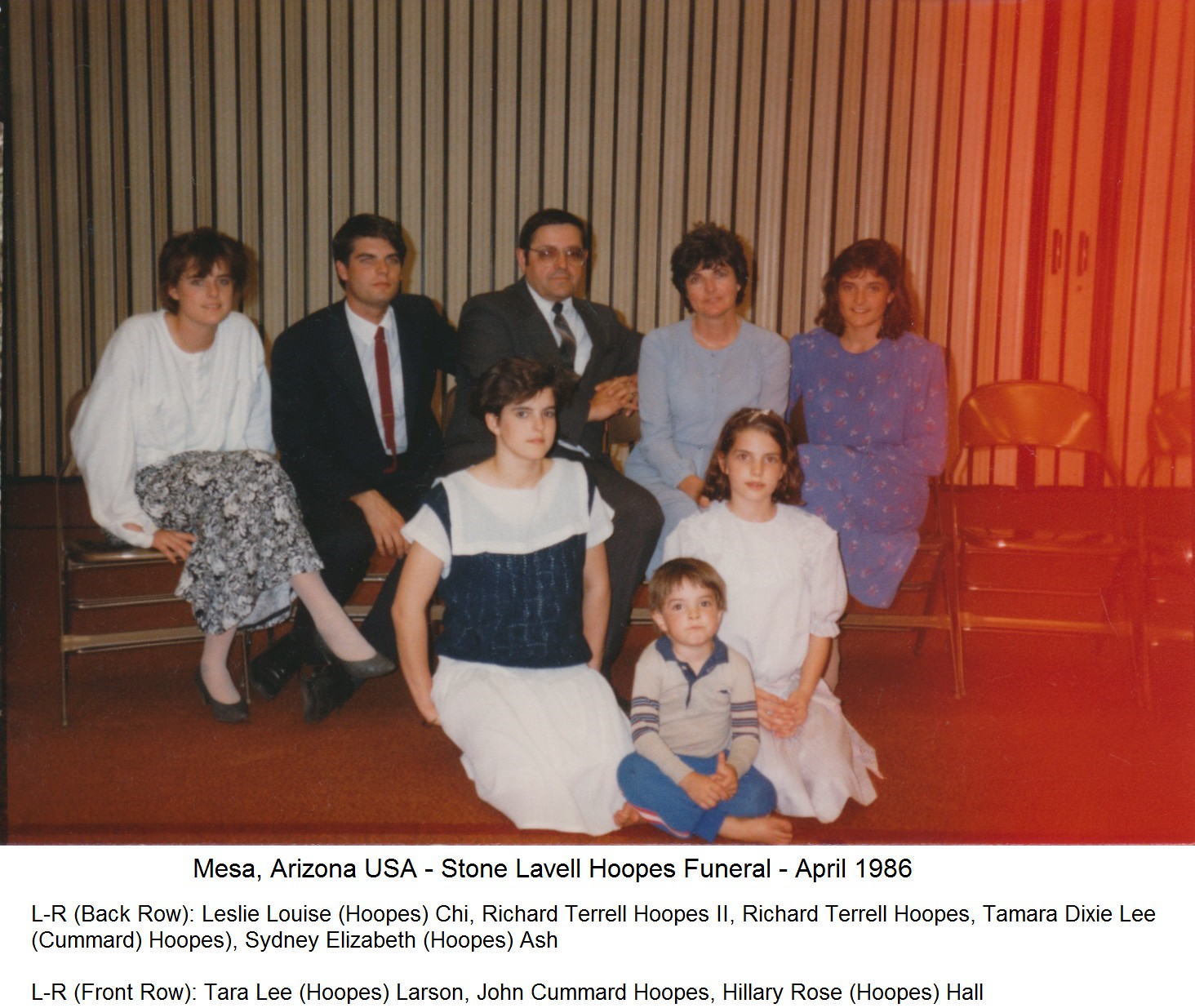This color photograph from April 1986 depicts eight individuals at the funeral of Stone Lavelle Hoopes in Mesa, Arizona, USA. The image features a group seated in two rows with a brown paneled wall in the background, typical of event spaces that can be divided. The photograph has a noticeable red tint on the right side, possibly due to film exposure issues.

In the back row, seated on metal folding chairs, are five adults dressed formally. From left to right:
- Leslie Louise Hoopes Chai, in a white blouse and black-and-white skirt.
- Richard Terrell Hoopes II, wearing a black suit with a red tie.
- Richard Terrell Hoopes, an older man in a gray suit with glasses.
- Tamara Dixie Lee Cummerd Hoopes, in a light blue dress.
- Sydney Ella Elizabeth Hoopes Ashe, in a medium blue dress with a white dotted pattern.

In the front row, three younger individuals are kneeling or sitting on the floor:
- Tara Lee Hoopes Larson, about 16 years old, in a dark blue and white outfit.
- John Cummerd Hoopes, a barefoot boy around three or four years old, wearing a gray shirt and blue pants, sitting cross-legged with a bemused expression.
- Hillary Rose Hoopes Hall, approximately 12 or 13 years old, in a white top and blue middle dress with brown shoulder-length hair.

The overall aesthetic of the scene, complemented by the dark orange-red carpeting, is indicative of the 70s or 80s era, with a slightly hazy quality to the photograph.